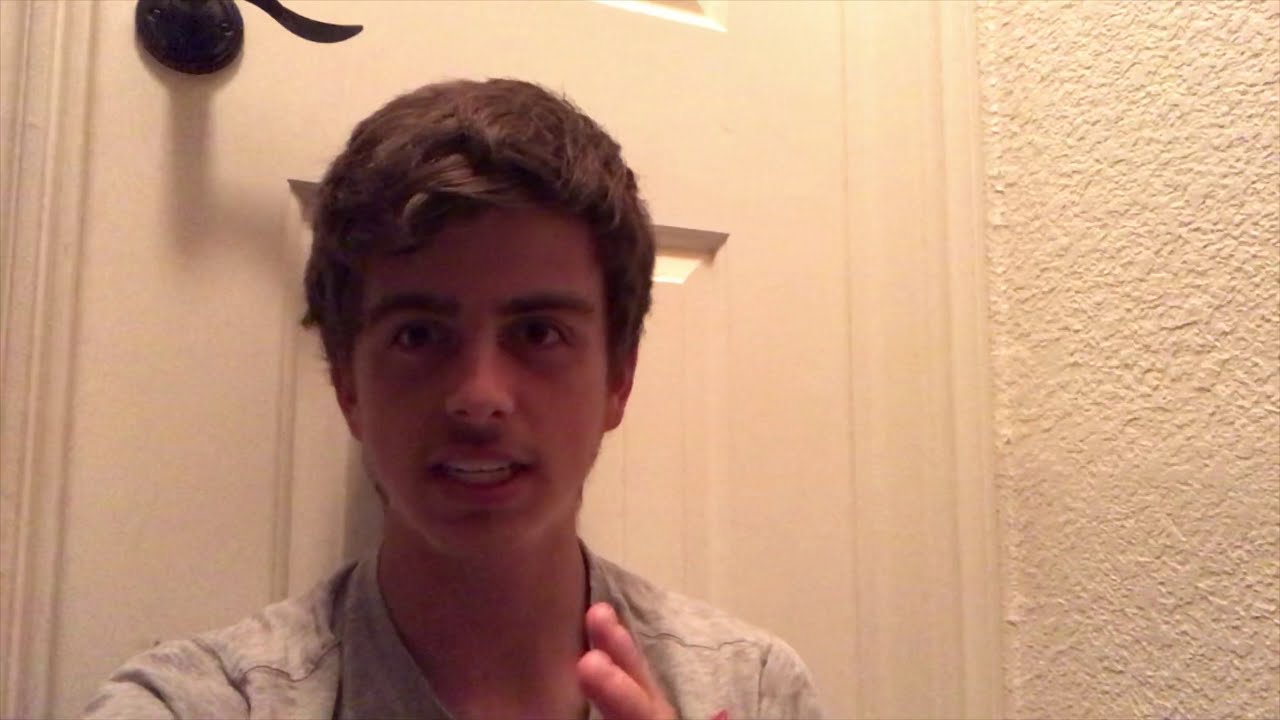The image depicts a Caucasian male with short, brown hair styled with a slight curl to the side and thick eyebrows. He appears to be taking a selfie in a bright room, with his white, eggshell-colored door visible behind him, featuring a black handle and latch positioned above his head. He is dressed in a gray t-shirt and has a faint goatee. His mouth is slightly open, showing both rows of his teeth, suggesting he might be speaking or explaining something. His left hand is partially raised and visible in the frame. To his left, there's a textured, off-white wall, adding a sense of depth to the setting. The overall image quality is low, hinting it might have been taken in dim lighting.